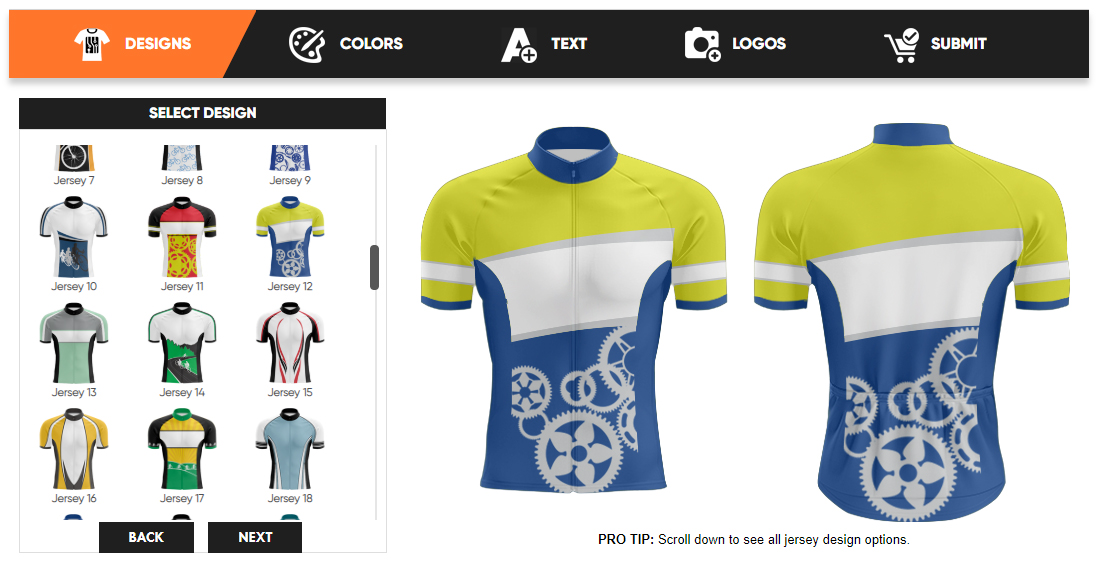The webpage is an e-commerce platform showcasing sports jerseys with a highly detailed design layout. At the top of the page is an orange navigation bar featuring a white and black shirt logo next to the word "Designs." Adjacent to this, within a black background, are tabs for "Colors," "Text," "Logos," and a "Submit" button, symbolized by a shopping cart icon. On the left sidebar, users can scroll through and select various jerseys, numbered from 7 to 21. 

The image prominently displays a highlighted jersey in the center-right section, featuring a striking yellow and blue color scheme with intricate gear designs on the lower part of the shirt. The jersey is showcased on a headless and armless mannequin, presenting both the front and back views. Below the jersey, there's a pro tip advising users to scroll down to view all available jersey design options. Additionally, the page includes "Back" and "Next" buttons on the left side, both with a black background and white font.

The website's overall style is sleek and user-friendly, designed to provide a seamless experience for customizing sports jerseys, reflecting a sophisticated web design interface.